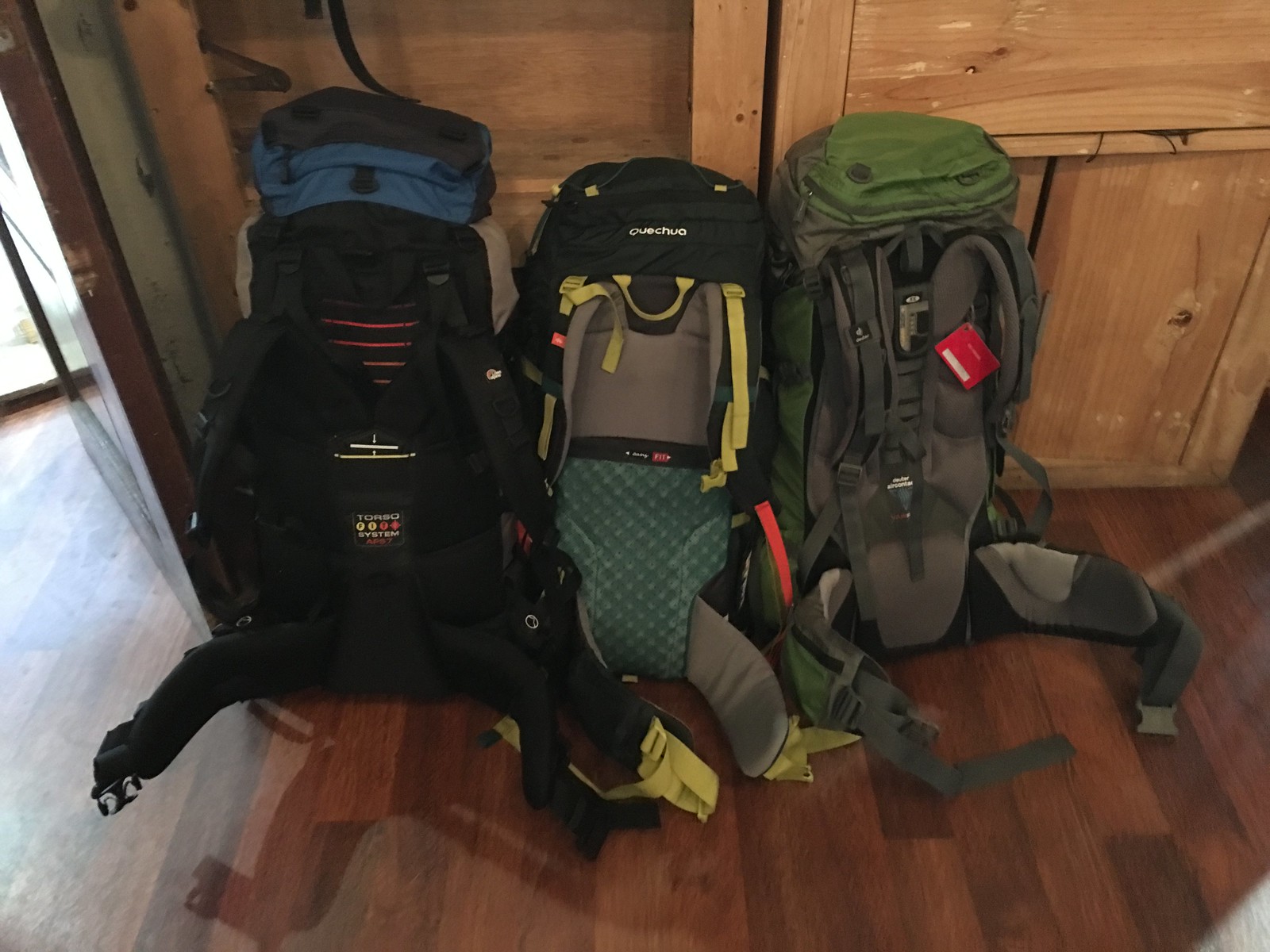This photograph captures a close-up view of three large, outdoorsy backpacks leaning against a wooden wall in what appears to be the entrance of a house. The scene is warmly lit with daylight streaming in from the left side through an open door. The floor beneath the backpacks is hardwood with a reddish hue, complementing the natural wooden wall against which the backpacks are placed. Each backpack dominates its section of the frame with distinctive details: 

- The backpack on the left is predominantly black with a blue top and features a waist strap for added support.
- The central backpack is a multicolored combination of green, gray, and a black top, adorned with a yellow strap detailing and a functional design that includes mid-body straps.
- The rightmost backpack is primarily a mix of khaki green and gray, featuring green accents at the top and a red business tag hanging from one of its straps.

The backpacks, which resemble those used for long hikes, are neatly positioned with their straps facing outward, showcasing their utilitarian features designed for serious trekking.